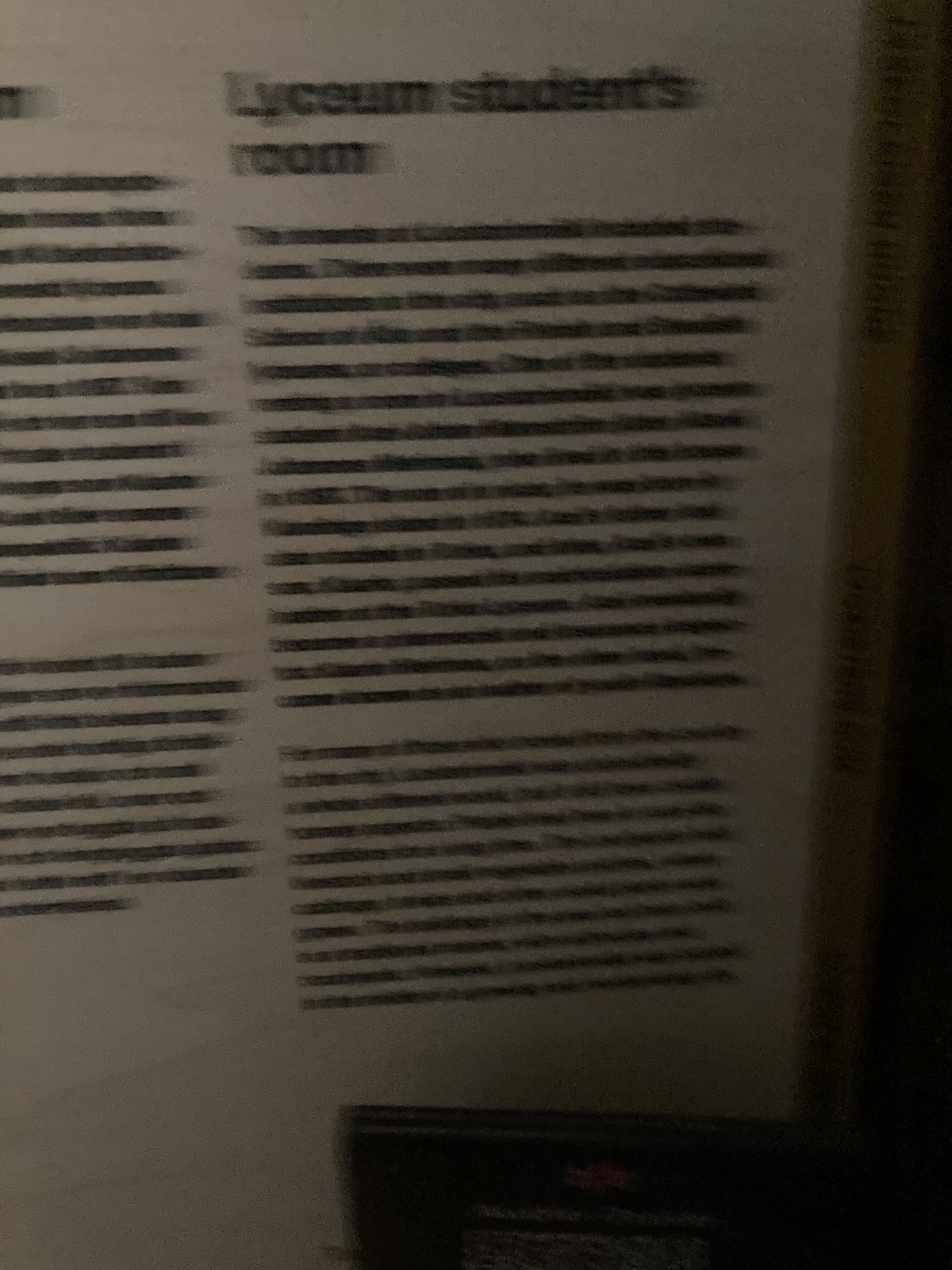The image features a dimly lit and blurry photograph of a sign or a page from a book. The text appears in black letters on a white background and is organized into two columns filled with numerous small, illegible words due to the blur. The top of the right column displays the text "Lyceum Student's Room" in a larger, more readable font. Toward the bottom right corner of the page, there is a very dark and shadowy area, almost obscuring this portion completely. The lower edge and the right side of the photo are enveloped in darkness, adding to the overall obscurity of the scene.